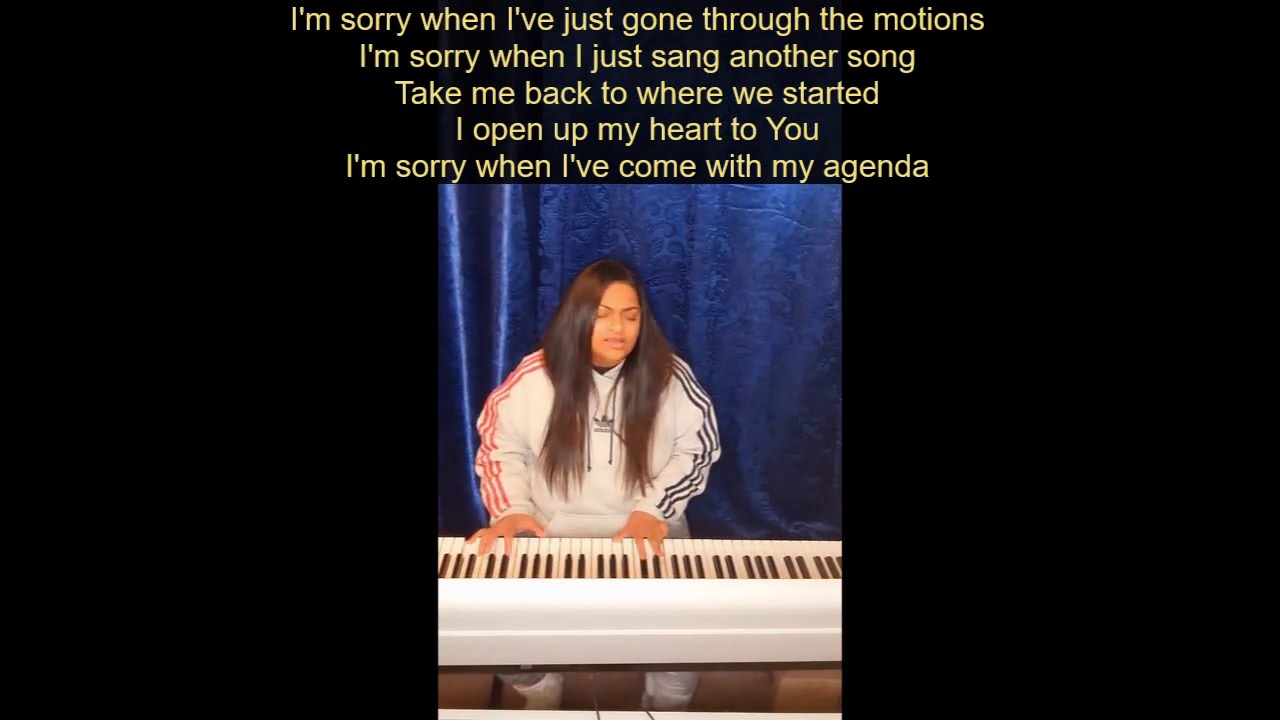In this image, a tan-skinned woman is sitting at a white keyboard piano with both black and white keys, positioned directly in the center towards the bottom of the frame. She is wearing a white shirt with the Adidas logo in black on the front, along with red stripes down her right sleeve and black stripes down her left sleeve. The woman's long, dark brown hair flows down almost to her hands, and she is seen with her eyes closed, suggesting she is deeply immersed in her performance. Only a portion of her legs, clad in white boots, are visible below the keyboard. Behind her hangs a blue curtain, adding depth to the dark background which also has significant black space. Centered at the top of the image is white text that reads, "I'm sorry when I've just gone through the motions. I'm sorry when I just sang another song. Take me back to where we started. I open up my heart to you. I'm sorry when I've come with my agenda." This text suggests the setting might be from a music video or screenshot, where the lyrics are displayed.